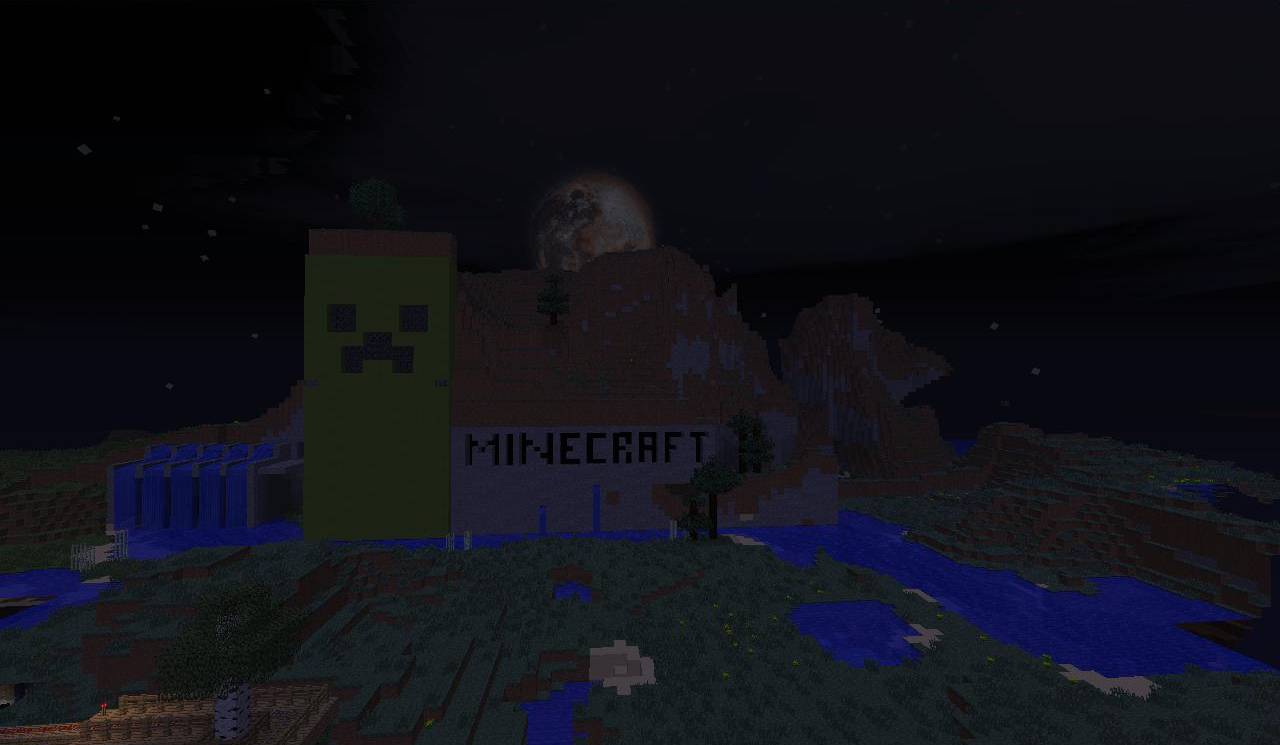The image is a screenshot from the popular game Minecraft, characterized by its iconic pixelated aesthetic. Dominating the center of the image is the word "Minecraft" in bold black font. Adjacent to this text on the left side is a three-dimensional rectangular block, likely representing wood, featuring a pixelated black frowny face on its surface. Below these elements, there is a pixelated depiction of Earth, with discernible green and blue regions that suggest landmasses and oceans, although stylized and distorted in the Minecraft manner. In the background, a depiction of the moon is faintly visible amidst an overall dark, black backdrop, creating a night-time scene. The entire composition is imbued with the signature blocky and pixelated texture synonymous with Minecraft, with Earth displayed at the bottom and the Minecraft title and frowny-faced block prominently floating above it.